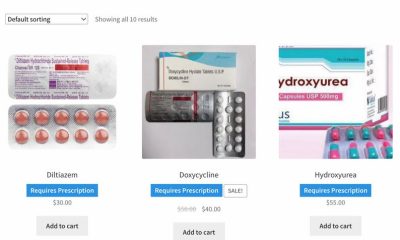The image displays a webpage for an online pharmacy. At the top of the page, there is a gray search bar set against a white background, accompanied by a dropdown menu labeled "default sorting." Above the product listings, a notice indicates "showing all 10 results."

On the top-left section, there's an image of a pill package. Although the text on the package is quite blurry, it features purple writing and a red banner beneath it. The packaging appears to be the type that holds pills in a silver aluminum foil, with visible indentations for each pill. The pack contains 10 red, round pills, arranged in two rows of five. The product name is "Diltiazem," followed by a blue banner stating "requires prescription" in white text. Below, the price is listed as $30. A gray "Add to Cart" button follows in black text.

To the right, there is another pill package on a gray background showing a clear depiction of a silver foil punch-out sheet filled with round white pills. The product is labeled "Doxycycline," an antibiotic. A blue banner with "requires prescription" is displayed in white, followed by a gray-outlined banner indicating "sale" in black. The price listed is $40 (though the first word preceding the price is too blurry to read). Below, another gray "Add to Cart" button is present.

Further to the right, another product image displays a blister pack of turquoise and pink capsules labeled "Hydroxyurea." Just below, a blue banner also reads "requires prescription" in white text. The price is marked at $55, and similar to the other listings, there is a gray "Add to Cart" button.